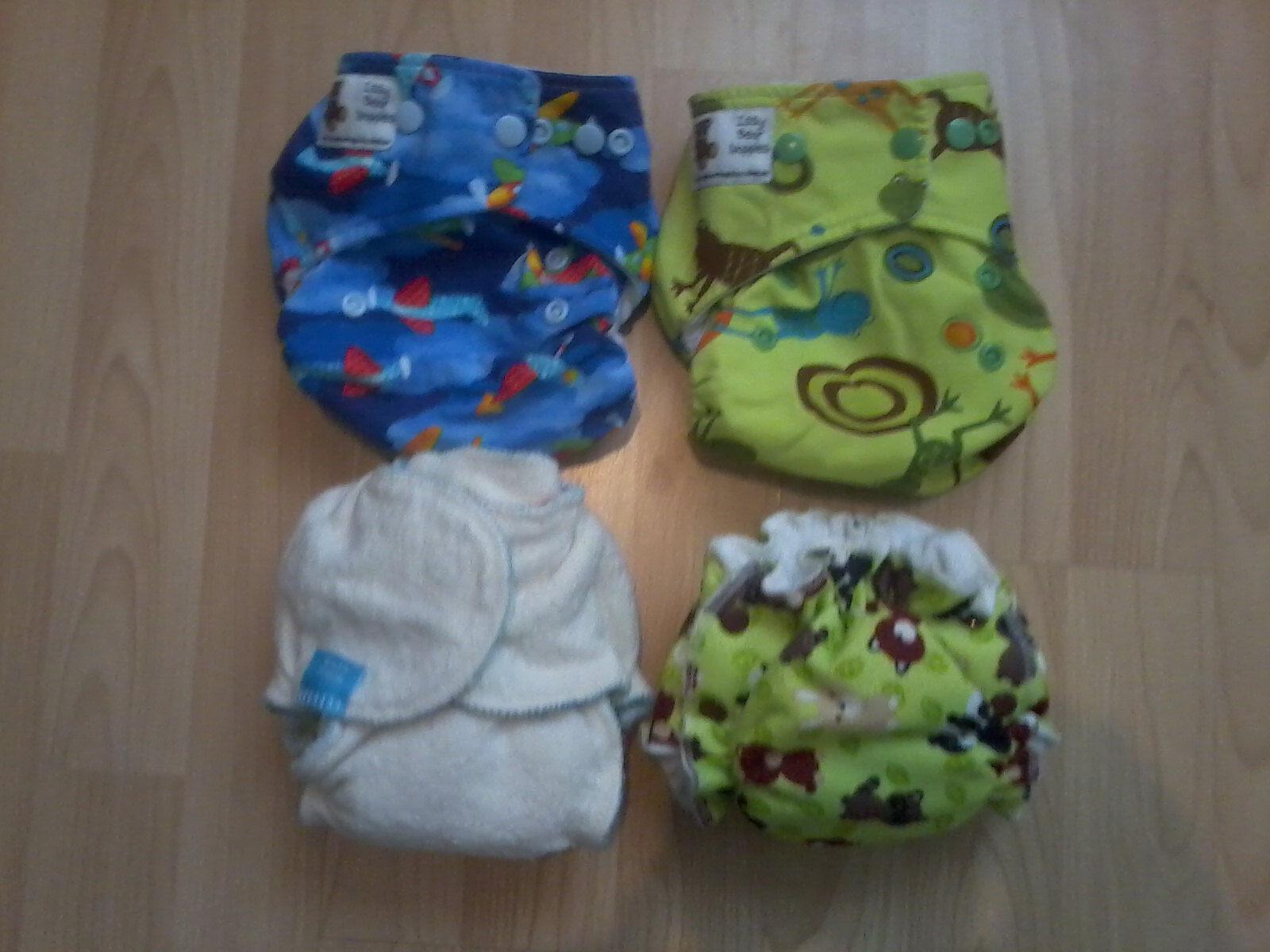The image depicts four baby garments laid out on a light brown wooden floor. Arranged in a square formation with two rows and two columns, each garment has distinct colors and patterns. The top left piece is a multicolored blue fabric adorned with an airplane motif in various hues, including red and darker blue, and features buttons. The top right garment is predominantly green with patterns incorporating circles, frogs, and possibly other designs in blues, browns, and oranges. The bottom left item is a simple gray or white fabric with a terry cloth texture, while the bottom right cloth is light green, showcasing illustrations of forest animals such as bunnies and bears, along with other colorful elements like reds, browns, and pinks. The image has a dim lighting and slightly blurry quality, making it somewhat difficult to distinguish the exact details and nature of the garments, which could resemble cloth diapers or similar baby attire.